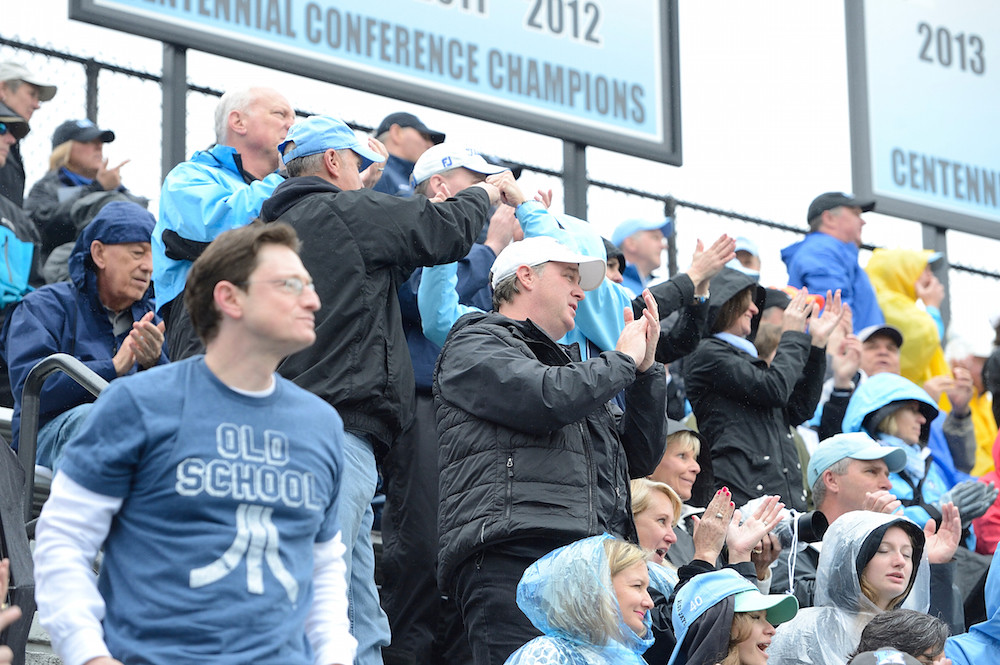A lively image depicts a crowd of fans packed into the stands at a sporting event. Despite the rain, their enthusiasm is palpable as many of them are clapping and cheering, likely in response to a recent play. The spectators are a mix of men and women, many donning rain gear such as rain jackets, rain hoods, and caps in varying colors, primarily blue and black.

Prominently featured in the bottom left of the image is a man with short brown hair and glasses, wearing a distinctive outfit: a blue t-shirt over a white long-sleeved shirt that reads "Old School." Nearby, to his right, stands another man in a white cap, dark shirt and pants, and a dark vest coat. In front of him, two women are visible; one wearing rain gear and the other in a cap, both facing to the right.

The stands are nearly full, and above them, two large blue billboards display partial texts: the left one reads "Conference Champions" and the right one, bearing "2013" and a truncated "Centennial.” The overall vibrant scene captures the community spirit and dedication of fans braving the weather to support their team.